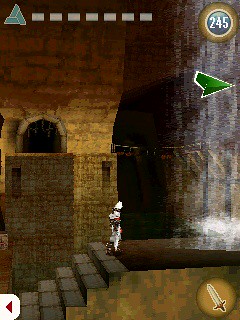This detailed screenshot captures the interior of a digital video game, appearing to take place inside a castle setting with gray stone walls, archways, and brownish-gray platforms. Central to the image is a stone staircase that ascends from a white block in the bottom left, marked with a red arrow, leading up to another level. A figure, presumably the player's character, enigmatic in appearance and somewhat dressed in white, is seen navigating these stairs. Positioned on the bottom right, there's a detailed depiction of a glowing brown sword with silver accents. In the center, a prominent pillar stands as a structural element. Surrounding this, a small four-cornered building features windows on either side, and a doorway or window-like opening at the far end. The top section of the screen displays a small triangle and seven rectangular dots, contributing to the game's interface elements. Furthermore, on the right side, there's a prominently glowing blue circle marked "245" in white, hinting at in-game statistics or status indicators. Finally, a green item, potentially an important in-game object or indicator, is also visible at the top right of the screenshot.